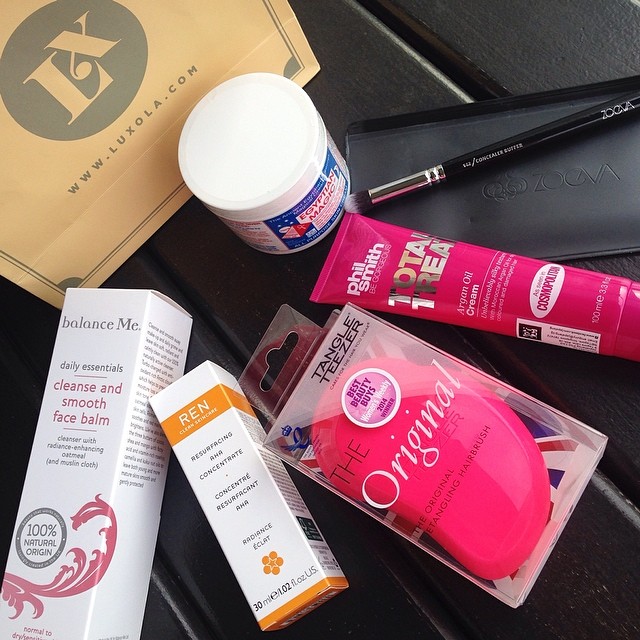The image displays an assortment of beauty and skincare products set against a black background. Prominently featured is a black pencil-like object with the words "Zova" in white, ending in a paintbrush-like brush. A brown box with the letters "LX" in brown, encircled by a black ring, along with the URL "www.lexsola.com" in black on its surface, is also present. Beneath this, a white tube with a blue front reads "Egyptian Magic" in red on a white background. Another box reads "balance me daily essentials cleanse and smooth face balm," with labels in black or gray letters. An adjacent item features an orange strip with the word "Ren," and below it phrases including "concentrate reassurance" in black letters, accompanied by five orange bubbles around a star. Two pink objects are visible, the topmost labeled "Phil Smith, Total Treat Argan Oil Cream" in white. Additionally, a white logo on the see-through package states "Cosmopolitan Best Beauty Buys 2014." The entire arrangement, signifying a collection of beauty products, appears to come from the website www.lexsola.com.